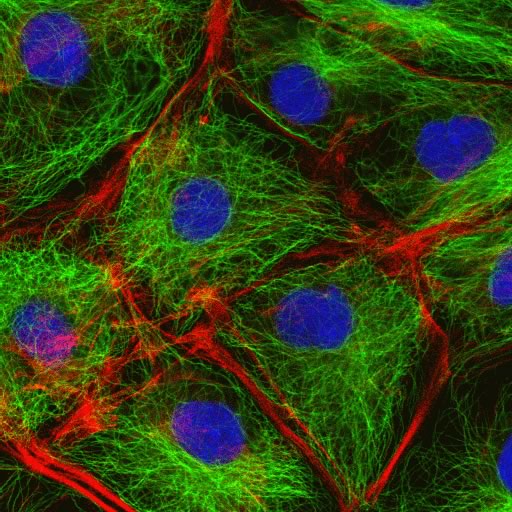This image appears to be a highly detailed and vibrant microscopic image, likely depicting a fabric or fiber structure. The predominant feature is a red netting that provides a structured, mesh-like background. Interwoven within this netting is a fibrous, tissue-like substance in green, adding texture and depth to the composition. Scattered throughout the image are several blue dots, reminiscent of tiny eggs, which seem to have been intentionally added. The rich colors—red, green, and blue—combine to create an abstract and visually appealing piece that exudes both structure and calmness. The red netting surrounds the green fibers, giving the image a sense of solidity and organization, while the blue dots provide a playful contrast. The intricate details and vivid colors make this image not only scientifically intriguing but also aesthetically pleasing, suitable for display as a piece of abstract art.